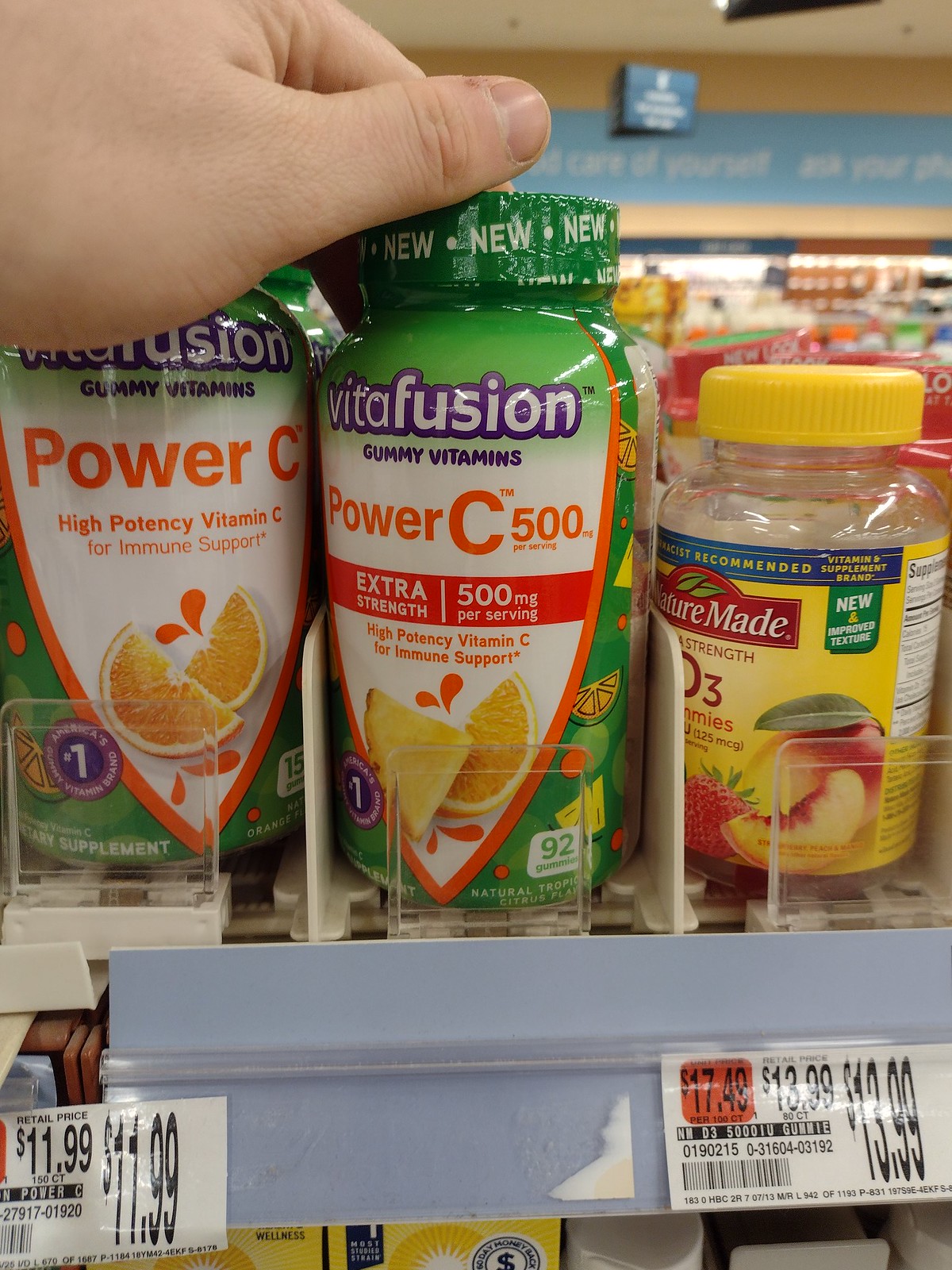A brightly lit interior of what appears to be a CVS store, showcasing a well-organized vitamin section. In the foreground, a person is reaching for a bottle of gummy vitamins labeled "Fusion Gummy Vitamin Power C 500mg." The label highlights its high potency vitamin C for immune support. Adjacent to this bottle, there are similar vitamins, including an "Extra Strength" variant indicated by a red banner, and a "D3 Strength Gummy" with fruit flavors. Price tags are clearly visible, with the selected gummy vitamins priced at $11.99, not currently on sale. Additionally, the background captures a variety of other health-related products neatly displayed on the shelves.